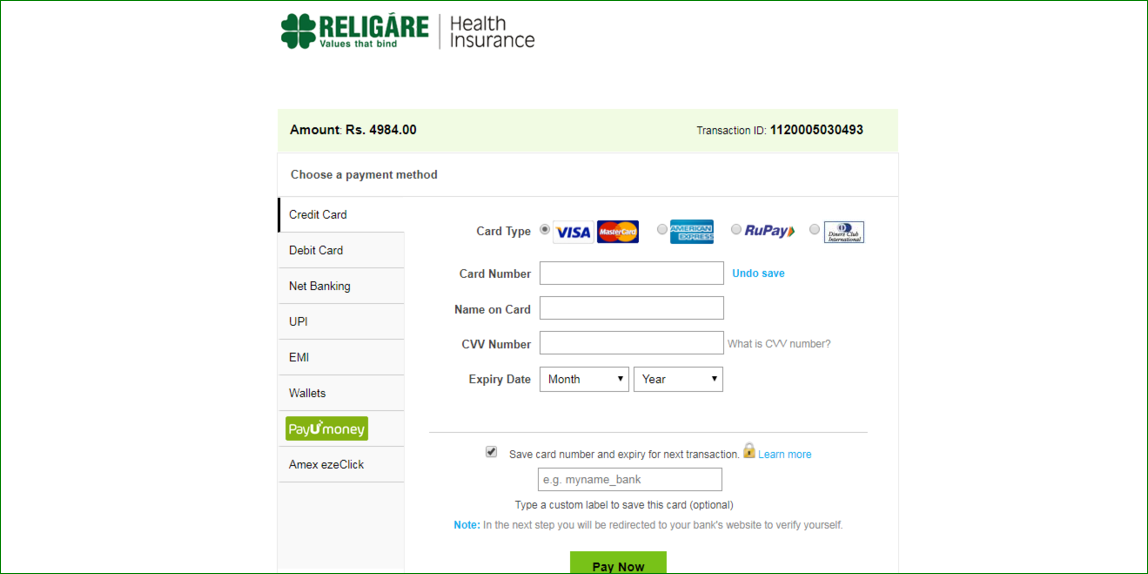This is a detailed screenshot from a website titled "Relagare Values That Bind Health Insurance." The title is prominently displayed in green font, and to its left is a four-leaf clover logo. The website features a predominantly white background, with one section highlighted in light green.

In the light green section, it details the "Amount of Risk" as "4984.00" and provides the "Transaction ID: 1120005030493." Beneath this, the instruction "Choose a Payment Method" is followed by a list of available options: Credit Card, Debit Card, Banking, UPI, EMI, Wallets, PayUMoney, Amex, and EasyClick. Presently, the "Credit Card" option is selected.

Within the "Credit Card" selection, users can choose between various card types: Visa, MasterCard, American Express, RuPay, or another type (the font is too small to identify the name). Currently, either Visa or MasterCard is selected. 

The section then prompts the user to enter their card details, including the card number, name on the card, CVV number, and expiry date. At this stage, these fields are blank. Adjacent to the CVV number field, there is a clickable question mark icon for users needing clarification on what a CVV number is.

Below these fields, there is an option to "Save Card Number and Expiry for Next Transaction," which is already checked, alongside an option to "learn more." Further down, there is a field for a custom label to save the card, suggested as "e.g., My Name_Bank," though this is optional. 

A note informs users that in the next step, they will be redirected to their bank's website to verify their account. Finally, at the very bottom, centered and within a green rectangle, is the "Pay Now" button.